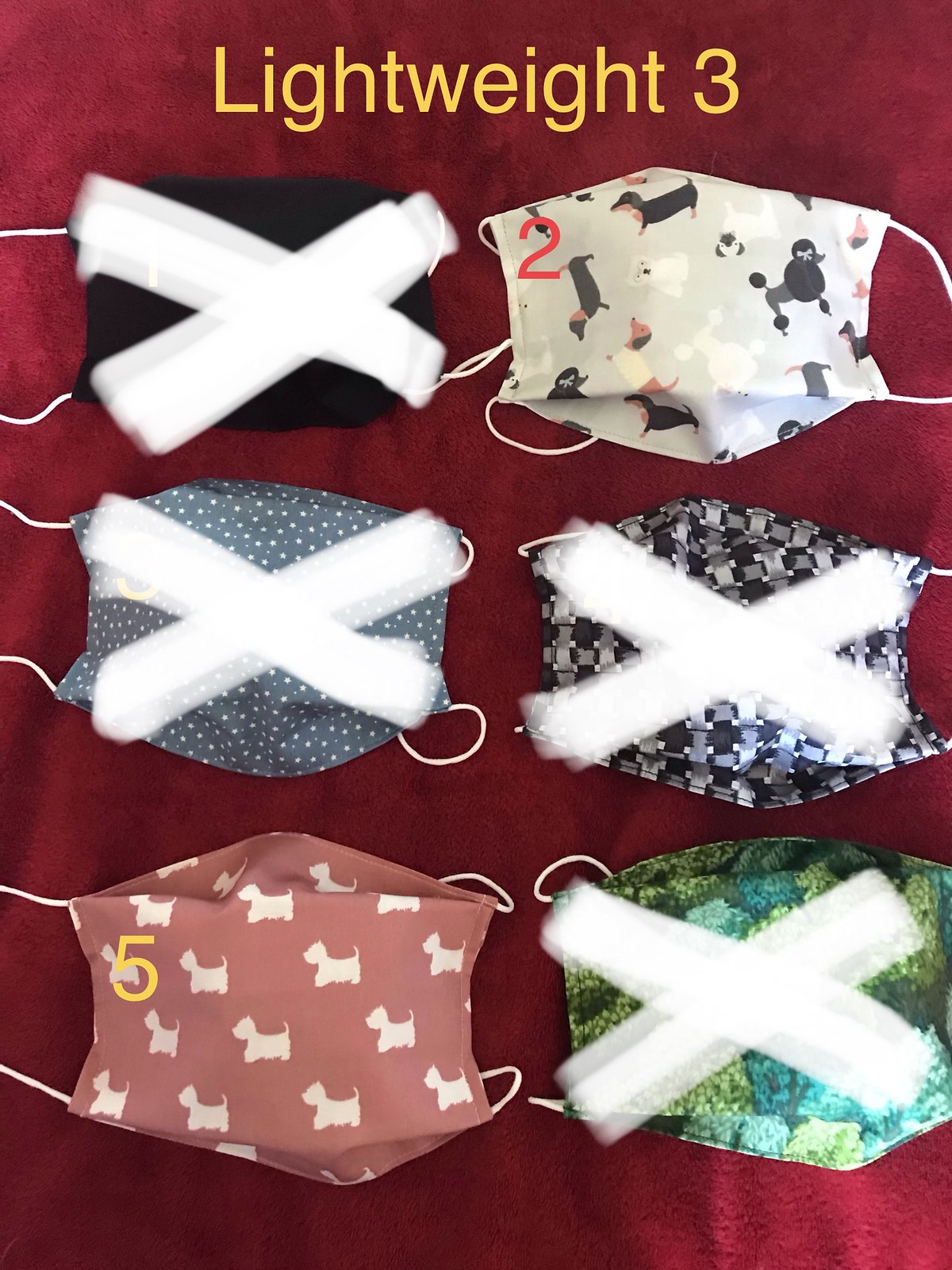The webpage showcases a set of six face masks displayed on a rich red velvet background with the text "Lightweight" written in yellow at the top, along with the number three. Out of the six masks, four are marked with a white X, indicating they are not available. The available masks include a light pink mask adorned with small white terrier dogs and a light-colored mask featuring various dog breeds, such as black and white poodles. The crossed-out masks are a solid black one, a blue one with polka dots, a black and white plaid mask, and a mask with a mix of light and dark green squares. Each mask comes with white elastic strings designed to go around the ears for a secure fit.